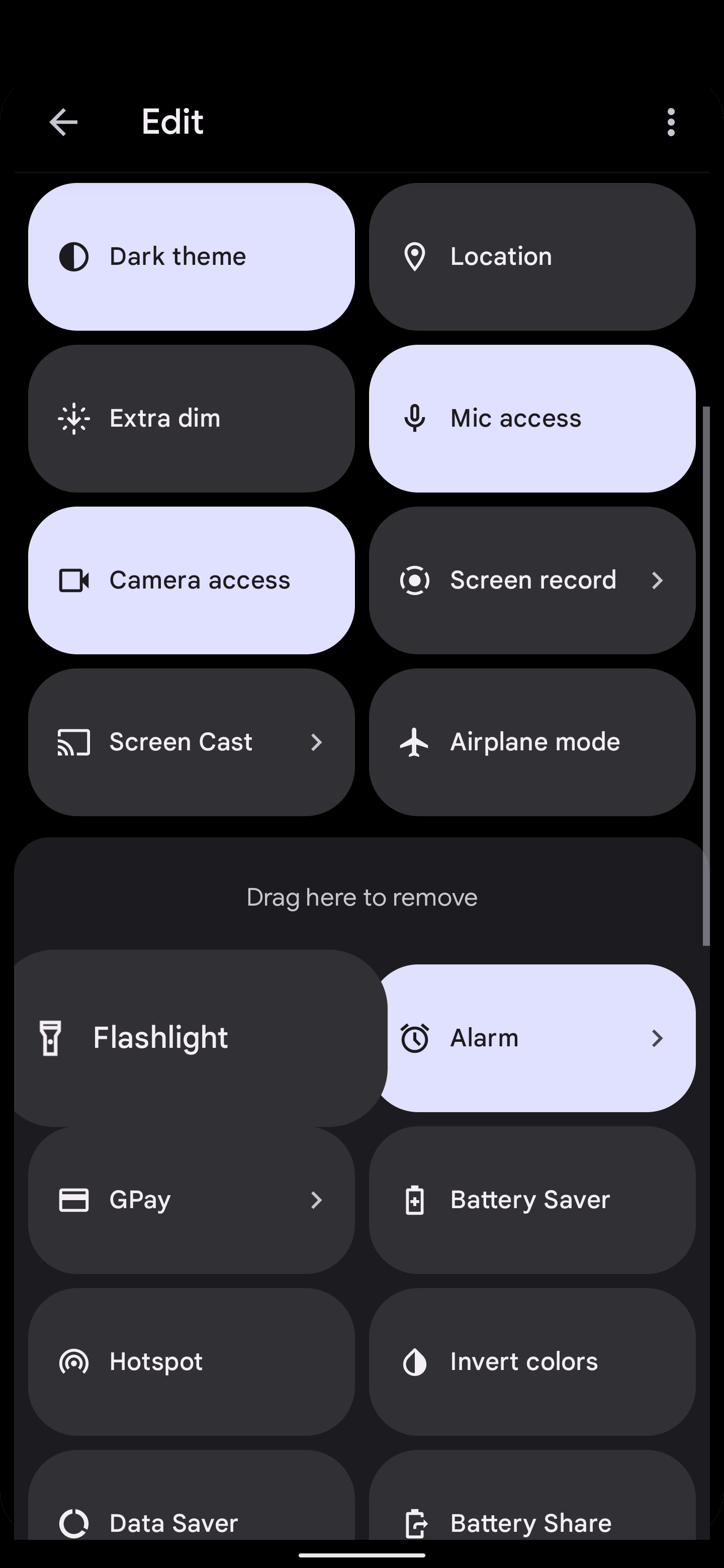This image appears to be a screenshot from a smartphone in portrait mode, predominantly characterized by a black background. The interface is segmented into various rectangular buttons with rounded corners displaying text. There are a total of 16 buttons arranged in two distinct sections: eight at the top and eight at the bottom, divided by a larger central rectangle with the directive "Drag here to remove".

The right side of the screen features a scrollbar, suggesting additional content that can be scrolled through. At the top, there's an "Edit" option in white text, flanked by a left-pointing arrow and three dots on the far right, indicative of additional settings or menu options.

The majority of the buttons are dark grey except for four that are highlighted in light grey: "Dark theme," "Mic access," "Camera access," and "Alarm." Each button contains accompanying icons, such as an alarm clock for the "Alarm" button and a flashlight for the "Flashlight" button. Furthermore, four buttons— "Screen record," "Screencast," "Alarm," and "GPay"—have an arrow on their far right, possibly indicating more options or settings upon selection.

Here's a detailed list of the buttons with their respective labels and icons:
1. Dark theme (Highlighted)
2. Location
3. Extra dim
4. Mic access (Highlighted)
5. Camera access (Highlighted)
6. Screen record (With arrow)
7. Screencast (With arrow)
8. Airplane mode
9. Flashlight
10. Alarm (Highlighted, with arrow)
11. GPay (With arrow)
12. Battery saver
13. Hotspot
14. Invert colors
15. Data saver
16. Battery share

Each button is designed with an intuitive icon representation to the left, enhancing user accessibility and understanding of each function.